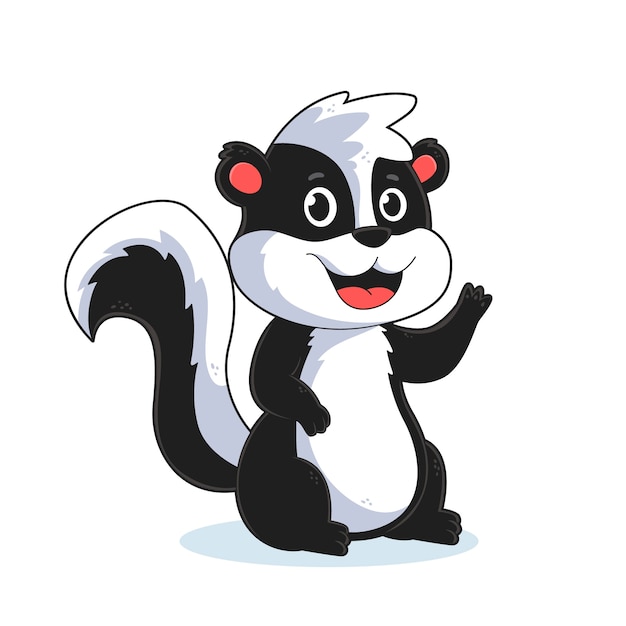The image is a detailed cartoon illustration of a skunk set against a completely white background. The skunk is seated on a small gray circle which serves as a kind of surface or shadow beneath it. With its left arm raised in a friendly wave on the viewer's right side, the skunk smiles warmly, displaying a pink tongue. Its eyes are large and white, encircled by black fur that extends across its face. The skunk’s ears are round and black with pink centers. A distinctive white stripe runs from its forehead to the back, splitting into three small triangular points atop its head. It has a black nose, and the rest of its face and belly are predominantly white, with hints of gray shading on the sides. The skunk's body is mostly black except for this white belly and a prominent white stripe on its bushy tail.